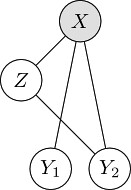This image features a simplistic and abstract formula, with no background details to provide context. Central to the composition is a gray circle labeled 'X'. To its left is a white circle marked 'Z', connected via a line to another white circle labeled 'Y2'. Above and slightly to the left of 'Y2', and connected to the gray 'X' through a line, is a third white circle labeled 'Y1'. All circles are outlined in black, and the overall arrangement of symbols suggests a specific, albeit unclear, pattern or relationship.